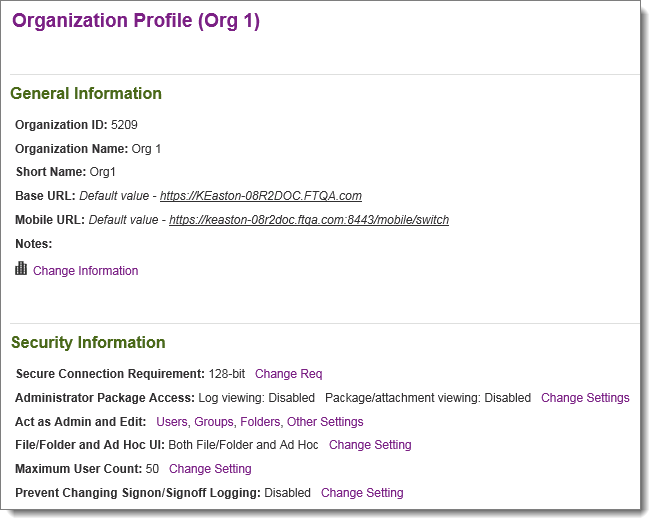Screenshot of Organization Profile

The screenshot captures the detailed profile of an organization. The title, "Organization Profile," is prominently displayed in purple. Below, the "General Information" section is highlighted in green. This section lists the following details in black lettering:

- Organization ID: 5209
- Organization Name: org1
- Short Name: org1
- Base URL: K Easton
- Mobile URL: K Easton-08R2Doc

In this section, there is also a space for "Notes," which is currently empty.

Proceeding further, "Change Information" is marked in purple. Next, the "Secure Information" section appears in green print, with all associated details listed in black:

- Secure Connection Requirement: 128-bit

Following this, another purple section labeled "Change Request" provides additional settings:

- Administrator Package Access: Log Viewing Disabled
- Package Attachment Viewing: Disabled

This is followed by "Change Settings" in purple, which includes the following privileges:

- Act as Administrator: Edit users, groups, folders, and other settings.
- File Folder and Ad Hoc UI
- Both File Folder and Ad Hoc

A separate "Change Setting" in purple indicates that the maximum user count is set to 50.

Another "Change Setting" in purple specifies:

- Prevent Changing Sign-on/Sign-off Logging: Disabled

This series of detailed sections concludes the profile summary.